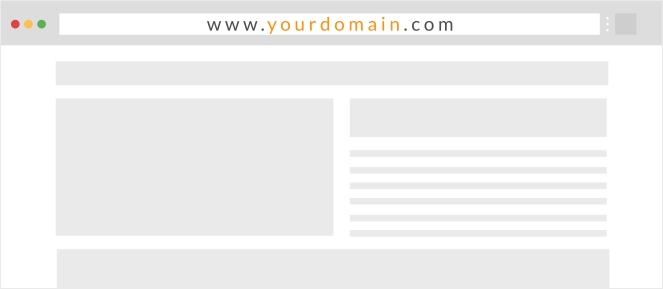This screenshot captures a minimalist design of a sample website. In the top left corner, it features the standard Apple OS buttons in red, yellow, and green, meant for closing, minimizing, and maximizing the screen. The main search bar at the top displays "www.yourdomain.com" with "yourdomain" highlighted in a striking yellow-gold color. 

Below the search bar, there are several placeholder elements set against a white background, indicating where content and interface elements would be positioned. This includes a long, light gray rectangular box, likely representing an input field or a banner. Directly beneath this, there is a section that suggests a photo placeholder, followed by slimmer lines that mimic header text and additional lines indicating where body text would appear. A larger, partially obscured box at the bottom suggests a prominent content area.

Overall, the screenshot showcases the structural layout without any actual text or images, providing a clear and organized blueprint for where various elements would be placed on the final webpage.